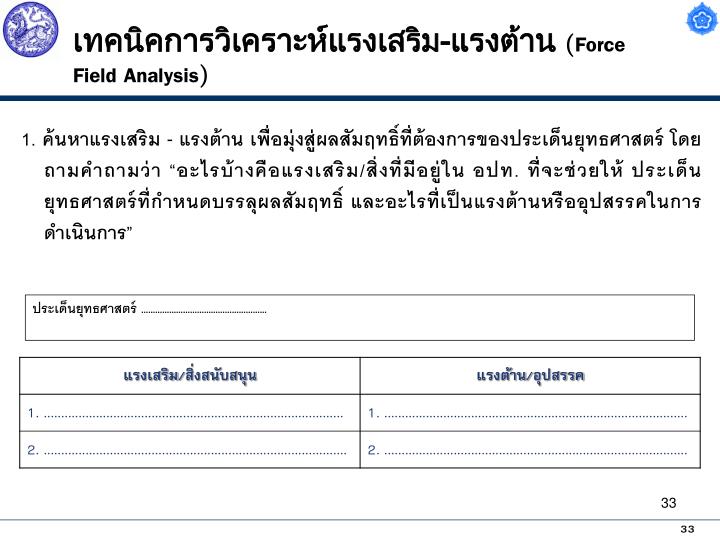The image depicts a primarily black and white form filled with foreign characters, likely in Thai. At the very top left of the form, there is a large blue emblem, possibly depicting an eagle, and to the right, a smaller purple medallion with a star inside. At the header, it features the English words "Force Field Analysis" in parentheses amid the predominant foreign text. Below the header, a thick black bar runs across the page. The top section includes a section labeled "1" for filling out information. Further down, the form is divided into two sections left and right, each numbered "1" and "2". The bottom right corner of the form displays the page number "33" in black text. The form’s overall design has black text on a white background.